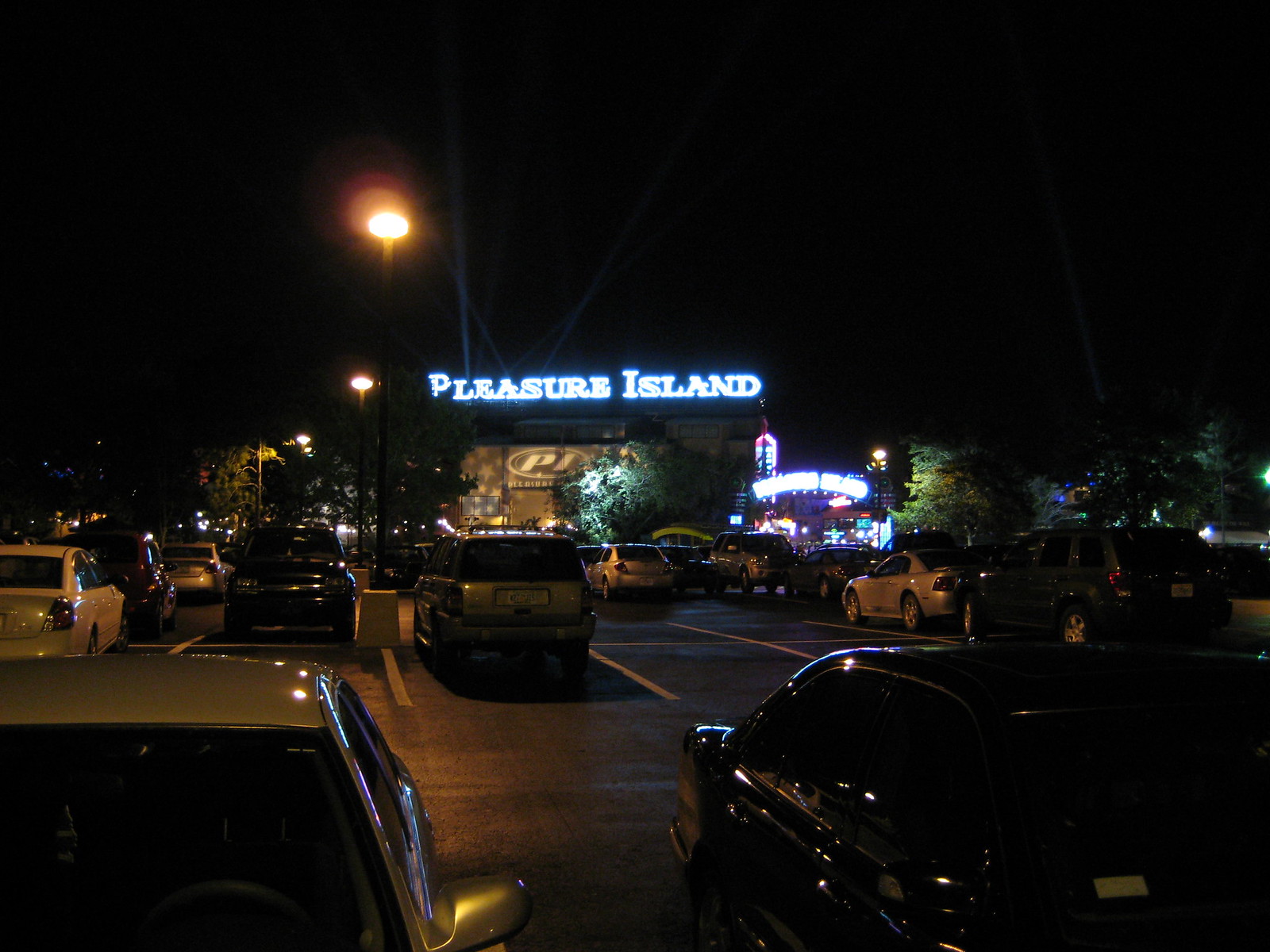This nighttime photograph captures a bustling scene featuring a wide road and an adjacent parking lot filled with a mix of sedans and SUVs. The black sky above is contrasted by various light sources that illuminate the area, including streetlights positioned in the median of the road. The road appears to have multiple lanes, possibly more than five, occupied by numerous cars, some parked and some moving. Dominating the background is a large, rectangular building adorned with a bright, glowing sign reading "Pleasure Island." This building, potentially a venue for nightlife activities, emits laser lights, adding to the vivid illumination of the scene. A brightly lit walkway lies to the right of this building, with green trees flanking either side of the entrance, enhancing the lively atmosphere. Overall, the image portrays a vibrant, busy nightlife setting with a significant amount of vehicular presence.